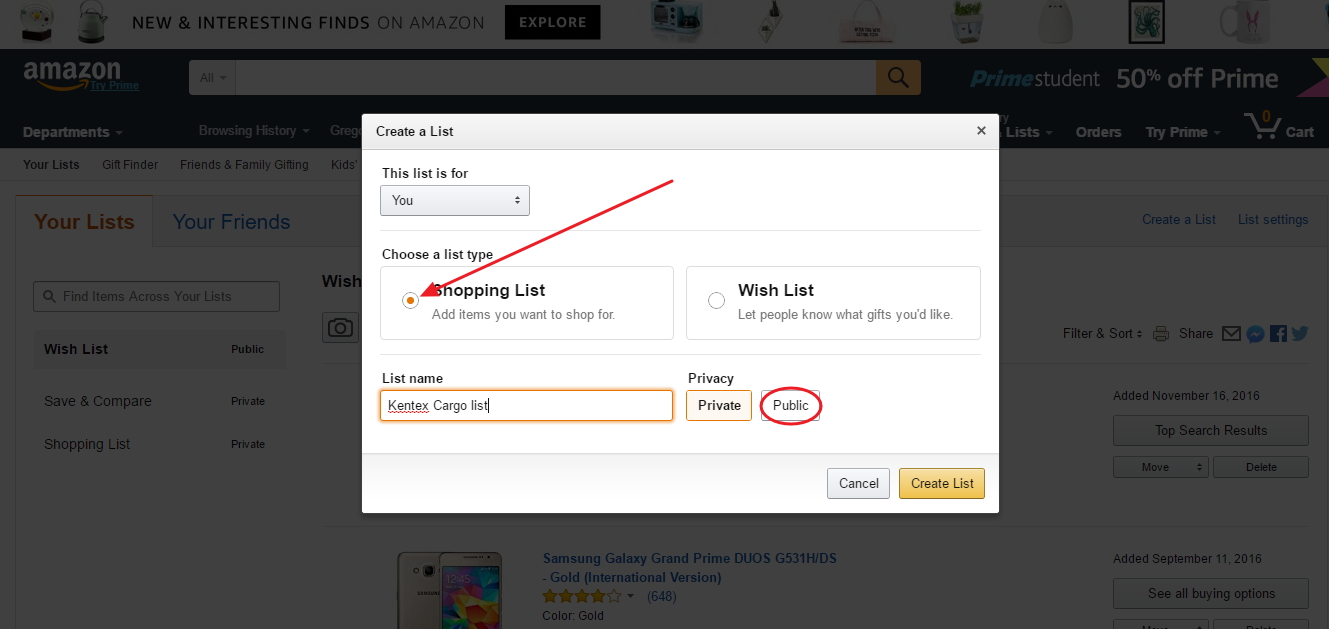The image showcases a screenshot of the Amazon website, with the background intentionally grayed out to obscure specific details. However, you can discern elements such as a Samsung Galaxy phone situated in the lower middle section and the main navigation headings across the top of the screen. The primary focus of the image is a prominent pop-up dialogue centered on the screen.

This large white dialogue features a light gray banner at the top, with the text "Create a List" positioned in the upper left corner. Below this, there is an editable field labeled "This list is for you," allowing for an alternative value to be specified from a pull-down list. 

Following this field is an option to choose the type of list, with two available choices: "Shopping List" and "Wish List." The "Shopping List" option is currently selected, and a large red arrow has been drawn, pointing at this option, presumably to emphasize its selection. 

Next, there is a section titled "List Name," containing an orange editable field where one can input the desired name for the list. Below this, there is a privacy setting option, which allows the list to be set as either "Private" or "Public." A red oval circles the "Public" option, indicating a suggestion to choose that particular privacy setting.

At the very bottom right of the dialogue, there are two buttons: a gray "Cancel" button and a yellow "Create List" button.